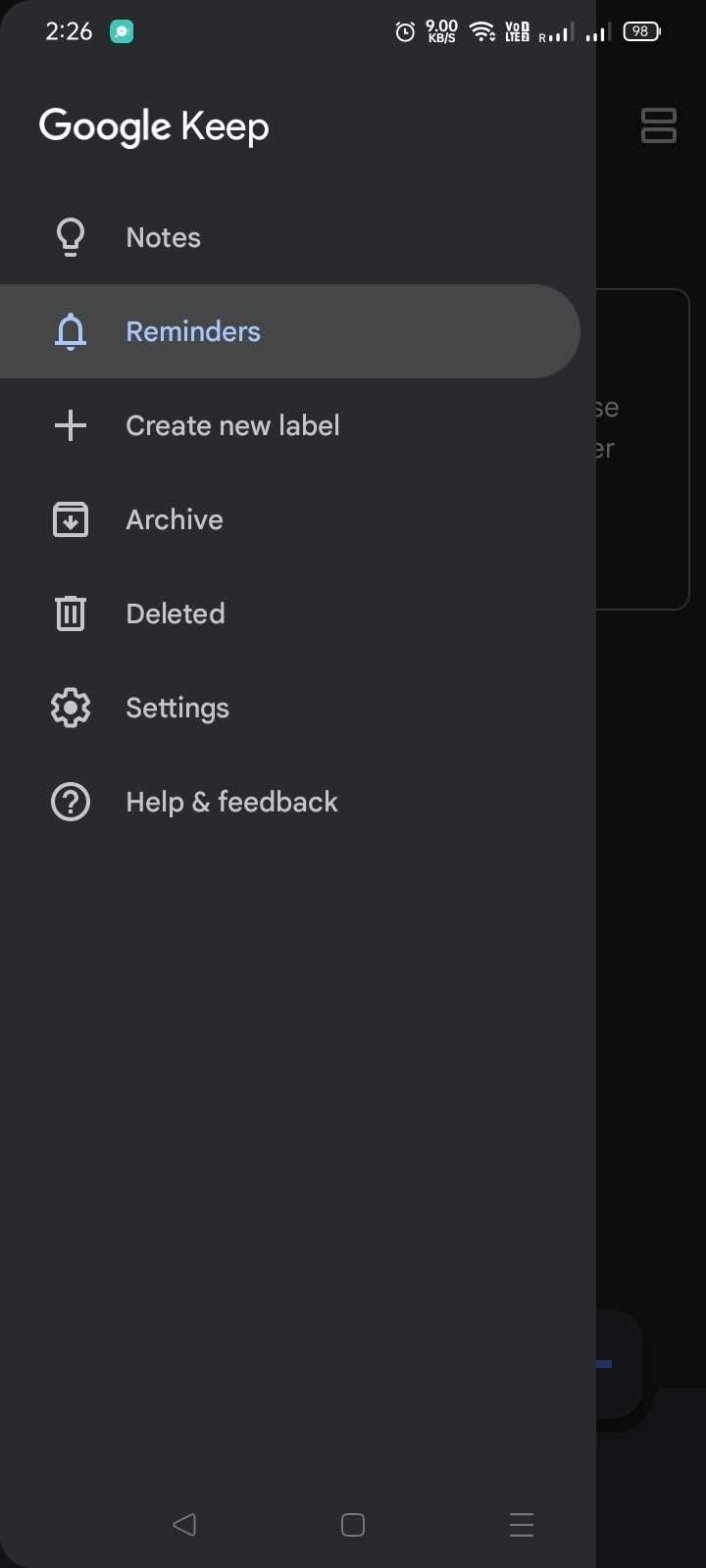The image features a close-up of a cell phone screen set against a dark background. In the upper left corner of the screen, the time reads "2:26." On the opposite upper right corner, various icons are displayed, including an alarm clock, an internet connection icon, and a battery icon showing "98".

Below these indicators, on the left side, there's a vertical column populated with text and icons. At the top of this column, the title "Google Keep" is prominently displayed. Directly below this title, an icon of a light bulb accompanies the text "Notes." Beneath the light bulb, an icon of a bell appears next to the text "Reminders," which is highlighted, indicating it is the currently selected tab. Moving further down, a plus sign is followed by the text "Create New Label."

Continuing downward, there is an icon of a rectangle with a downward-pointing arrow next to the label "Archive," followed by a trash can icon next to the text "Delete." Below them is a gear icon labeled "Settings," and further down, a circle with a white border encloses a white question mark, next to which the text reads "Help and Feedback."

At the very bottom of the screen, three icons sit against the dark background: an arrow pointing to the left on the left side, a square in the middle, and three horizontal lines stacked atop each other on the right.